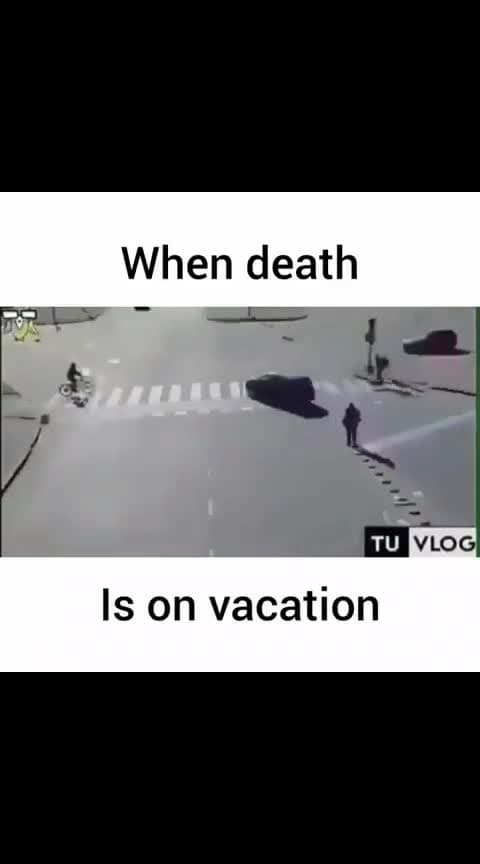The image resembles a screenshot taken on a phone, characterized by a vertical orientation. It features three horizontal rectangles on a solid white background. At the top and bottom of the screen are solid black rectangles framing the image. Between these two black bars is a central black-and-white photograph, bordered in white. The photograph captures an overhead view of what appears to be an intersection with a crosswalk marked by white dashed lines. 

Positioned at the upper part of the photograph in black text, it reads "When Death," while at the lower part it says "is on Vacation." In the picture, a bicyclist is seen riding through the crosswalk on the left side, and a vehicle is turning left on the right side. Behind the vehicle stands a man, creating a silhouette-like figure. There appear to be two vehicles approaching the intersection, one on the far right and another that is barely visible at the bottom of the photograph. A small traffic island or sidewalk with traffic lights is also noticeable between the vehicles on the right side. In the lower right corner of the image, the text "TUVLOG" is visible. The scene appears to highlight the precarious nature of the bicycles and pedestrian's positions amidst the vehicles.